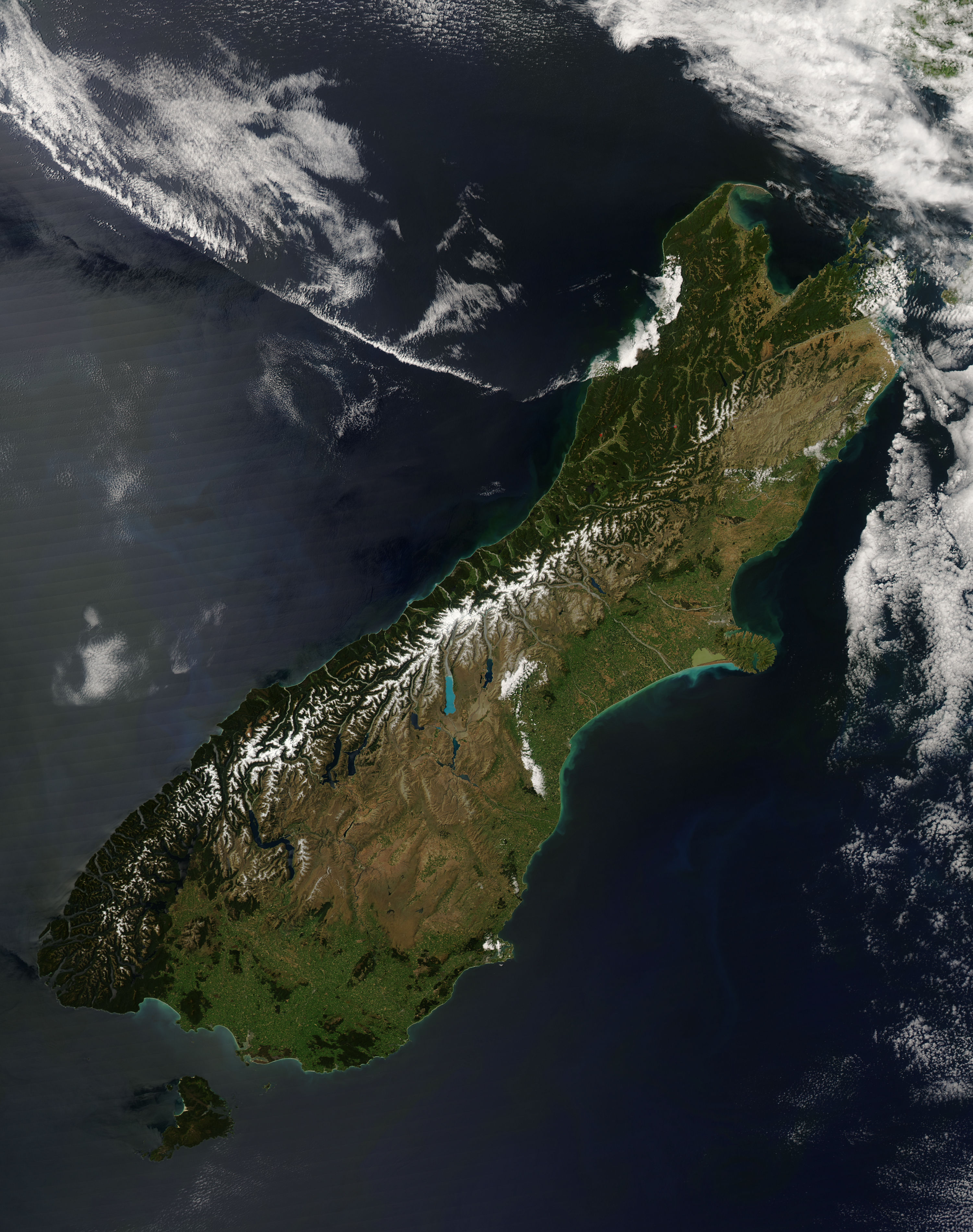This image is a detailed satellite photograph of the lower island of New Zealand, captured from orbit. The long, curved island stretches from the bottom left corner to the top right corner of the image. Surrounding the island is a vast expanse of navy blue ocean, punctuated by wisps of white clouds, especially noticeable along the right side and in the upper left corner. The island itself displays a rich palette of colors, including various shades of green, brown, and black, highlighting its lush landscapes and natural contours. There are no visible signs of civilization such as homes or roads, making the land appear untouched and pristine.